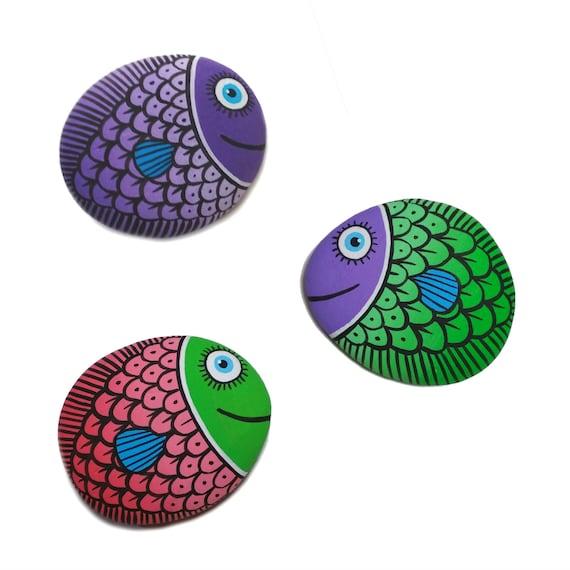This image features three egg-shaped stones painted to resemble fish, set against a white background. The stones are arranged in a loose triangle, with one in the top left corner, one in the middle right, and the last one on the bottom left. They are all facing towards the center, creating a sense of interaction among them.

The top left fish is primarily purple with purple scales, a matching purple face, and features a blue fin and a blue eye. The middle right fish, which faces left, has a green body with green scales, a contrasting purple face, a blue fin, and a blue eye. The bottom left fish, facing right, boasts a pink body with pink scales, a green face, a blue fin, and a blue eye. Each fish is adorned with a smiling black mouth, and they all seem to be joyfully engaging with one another, their expressions enhanced by small painted details like eyelashes.